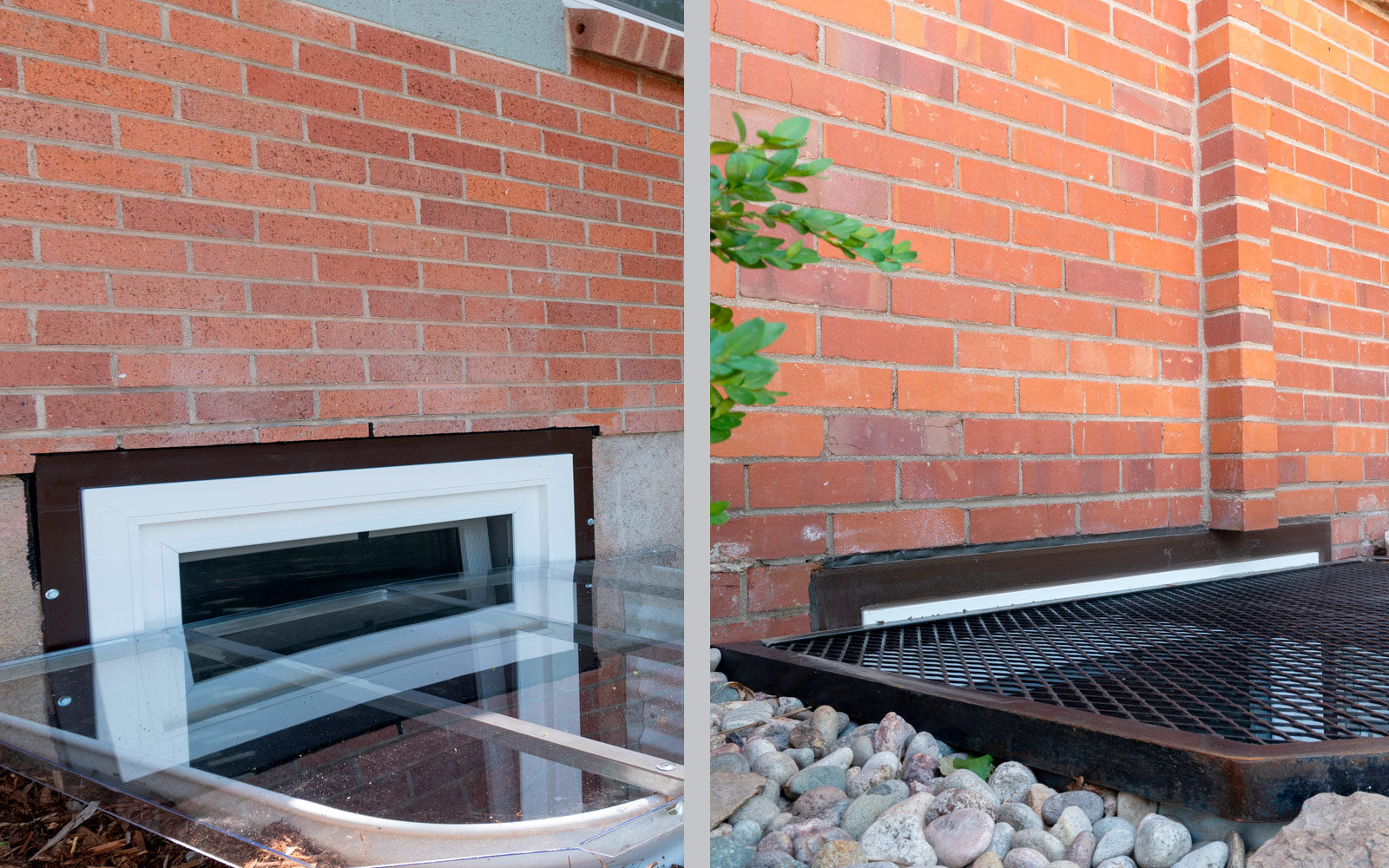This image displays a side-by-side comparison of two outdoor photographs taken in front of an orange and brown brick building with gray cement in between. Each photograph occupies one half of the image. Both pictures feature a rectangular window with a white-painted frame and a black border, situated near the ground level of what appears to be a basement or surface-level apartment. In the left-hand photograph, the ground below the window is covered with mulch, and there is a clear glass pane covering a U-shaped recess outside the window. In contrast, the right-hand photograph presents a dome-shaped black, ribbed metal grate resting on pebbled stones below the window, with a bush of green foliage partially visible. The brick wall in both images contains a vertical ridge, and both photos are taken under sunlight, suggesting they were captured at the same location but with different protective coverings for the window.